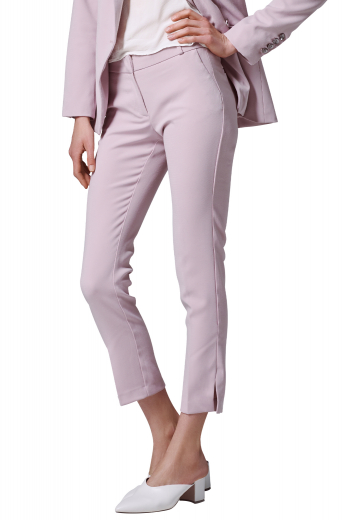This is a photograph of a woman wearing a stylish, coordinated lilac pantsuit. The suit includes a lilac blazer with four brown buttons on the left cuff and flared, ankle-length pants. She is also dressed in a white blouse and white mules with pointed toes and thick stacked heels. The image captures her from halfway up her torso to her feet. Her left hand is confidently placed on her left hip, while her right hand hangs relaxed by her side. The background is a simple white, ensuring the focus remains on her chic ensemble.